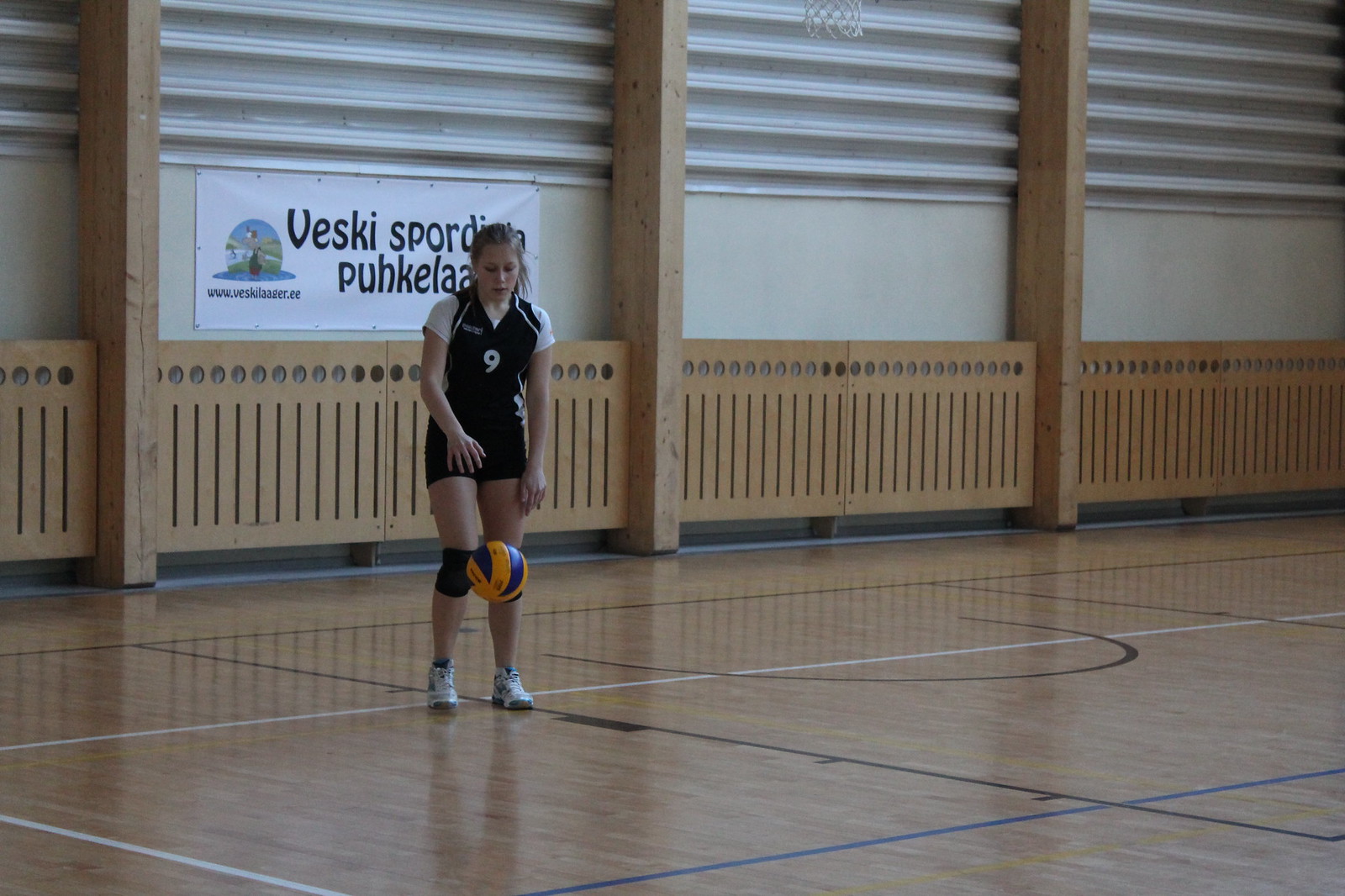Inside a white-walled gymnasium with a distinct wooden border featuring slots and circular designs at the top, a banner with partial text reading "VESKI SPORDI..." and "PUHKELA..." hangs prominently in the background. The scene centers on a fair-skinned preteen or teenage girl with light hair in a ponytail. She wears a black athletic uniform with short white sleeves, black shorts, white sneakers, and wraps on her knees. The number "9" is printed in white on her jersey. The floor beneath her is light brown, marked with black and blue lines. The girl is engaged with a yellow and blue volleyball, which is suspended midair as she prepares to either set or retrieve it. Her left arm is bent upwards, and her right arm is extended straight, underscoring her focus and determination in this athletic moment.